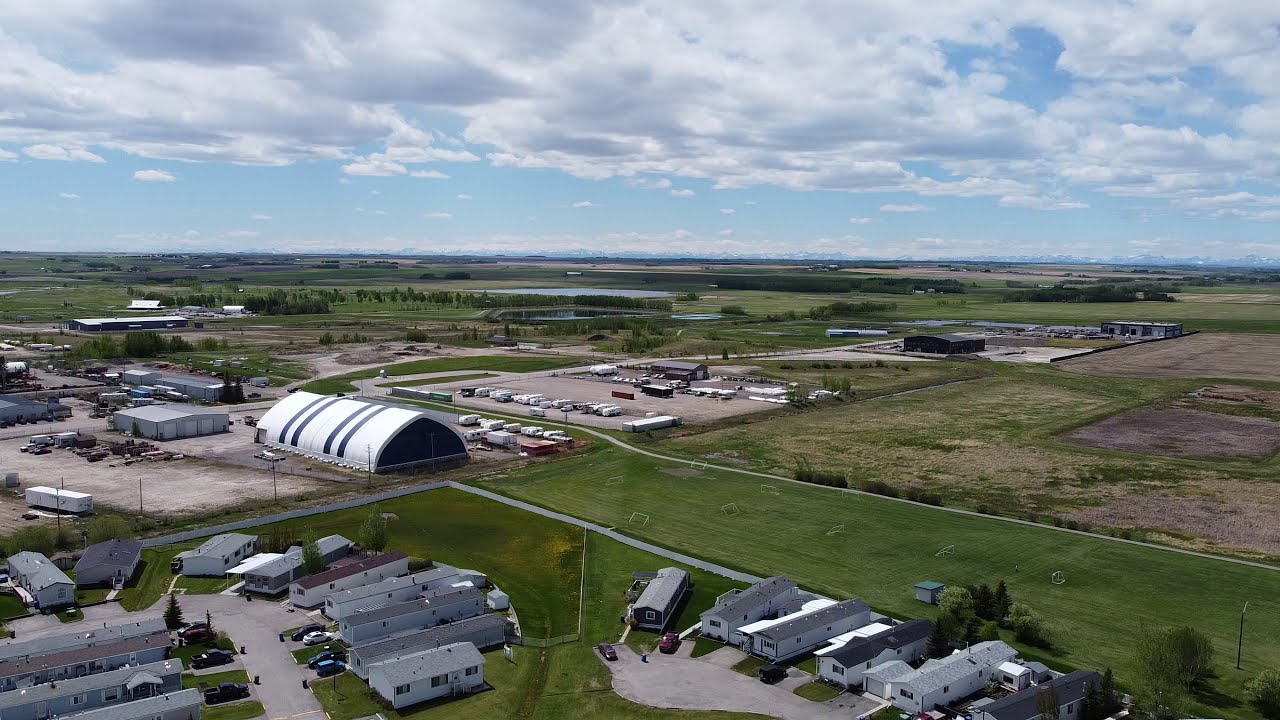This aerial photograph captures an expansive industrial center set in flat, middle American farm country. The primary feature is a sizable, bunker-shaped building, reminiscent of an airport hangar, characterized by its long, half-column design with four black stripes on its white roof. Surrounding the main structure are smaller, single-story, white and green buildings, including storage units and pre-manufactured homes, which are spread out across the landscape. The area is well-maintained, displaying neatly mown grasslands, with some patches extending towards the right side of the image. You can also spot several trailers and RVs near the main building, along with freight trucks and large paved areas with parked cars. There is a driveway weaving through the area, providing access to the various structures. In the background, fields, trees, and a couple of lakes are visible, accompanied by a river that adds a natural touch to the scene. The sky above is a beautiful blue, dotted with puffy white clouds, enhancing the serene yet industrious atmosphere of this setting.